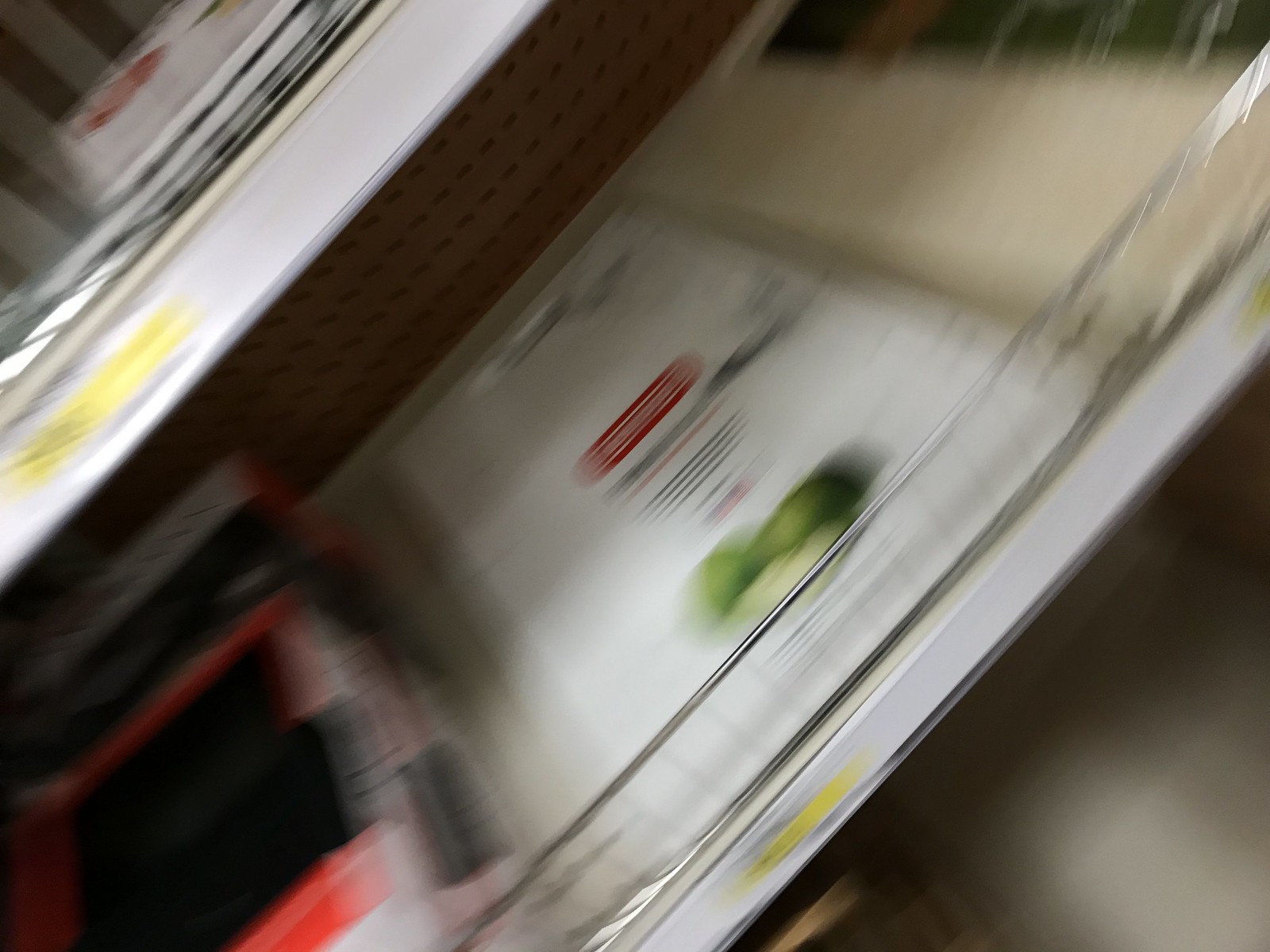The photograph depicts a set of shelves in a department store, captured in a slightly blurry manner. The two sections of white shelving feature yellow strips with black print, presumably price tags or shelf labels. A white cutting board with a red label and images of green fruit is discernible among the items on display. To the left of the cutting board, a red and white box with black accents stands out. A silver metal guardrail runs along the front, keeping the merchandise stable on the shelf.